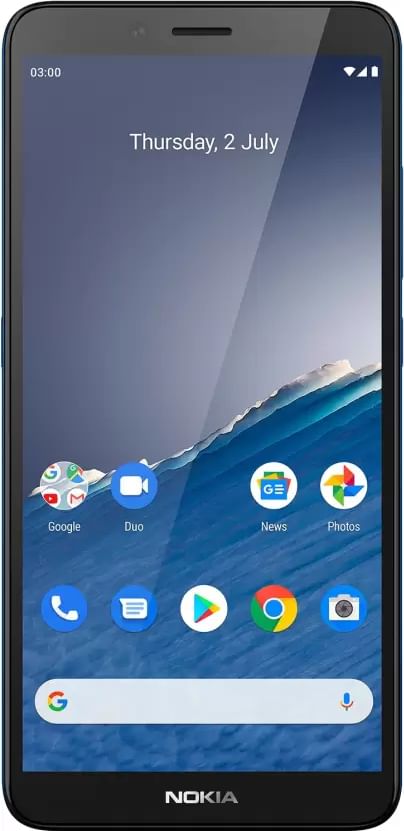The image depicts a complete view of a Nokia mobile phone. The phone features a distinctive black border encircling its edge, creating a thumb barrier. On the right side of the phone, there are two buttons positioned towards the upper section, while a single button is located on the left side, slightly above the midpoint. At the top center of the device, there's a narrow slit intended for audio output during calls, and a faintly visible camera to the left of this slit. The Nokia logo is displayed in a shiny white font on the black border at the bottom of the phone.

The screen showcases the main interface of an Android operating system. In the upper left corner, the current time is displayed, accompanied by status icons in the upper right. Centered just below the time, the date is indicated as "Thursday, 2nd July." The background image on the screen is an illustration of an ocean wave, radiating a subtle glow on the left side.

Near the bottom of the screen, two rows of app icons are visible. The upper row includes Google Duo, News, and Photos, while the lower row consists of icons for Phone, Google Play Store, Chrome browser, Camera, and Settings. Beneath these is a small white search bar with a Google logo on the left side and a microphone icon on the right, indicating the option for voice search.